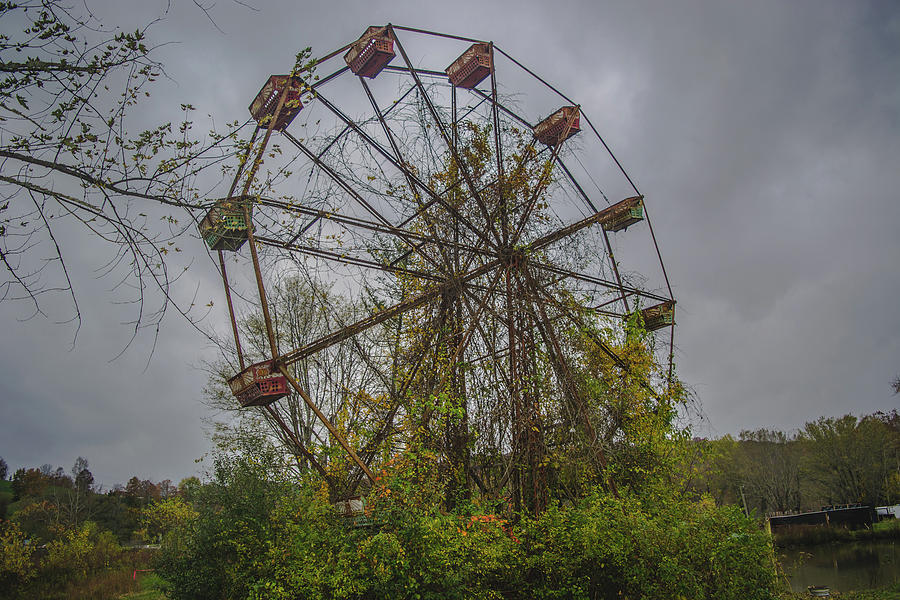This photograph captures an abandoned ferris wheel in an outdoor setting, depicted from a side view. The ferris wheel appears to have been out of service for a long time, evidenced by the overgrowth of vine plants and greenery that have taken over its structure. Some of the carriages, which are intact and display dark brown and green hues, are empty and contribute to the desolate atmosphere. On the ground, there are various plants and trees with green leaves and some flowers. The scene is further accentuated by a background of dense tree lines and an overcast sky filled with dark grey clouds, which adds to the sense of abandonment and decay. There are no signs of people, homes, or other rides in the vicinity, making the ferris wheel appear as a solitary relic left to be reclaimed by nature.